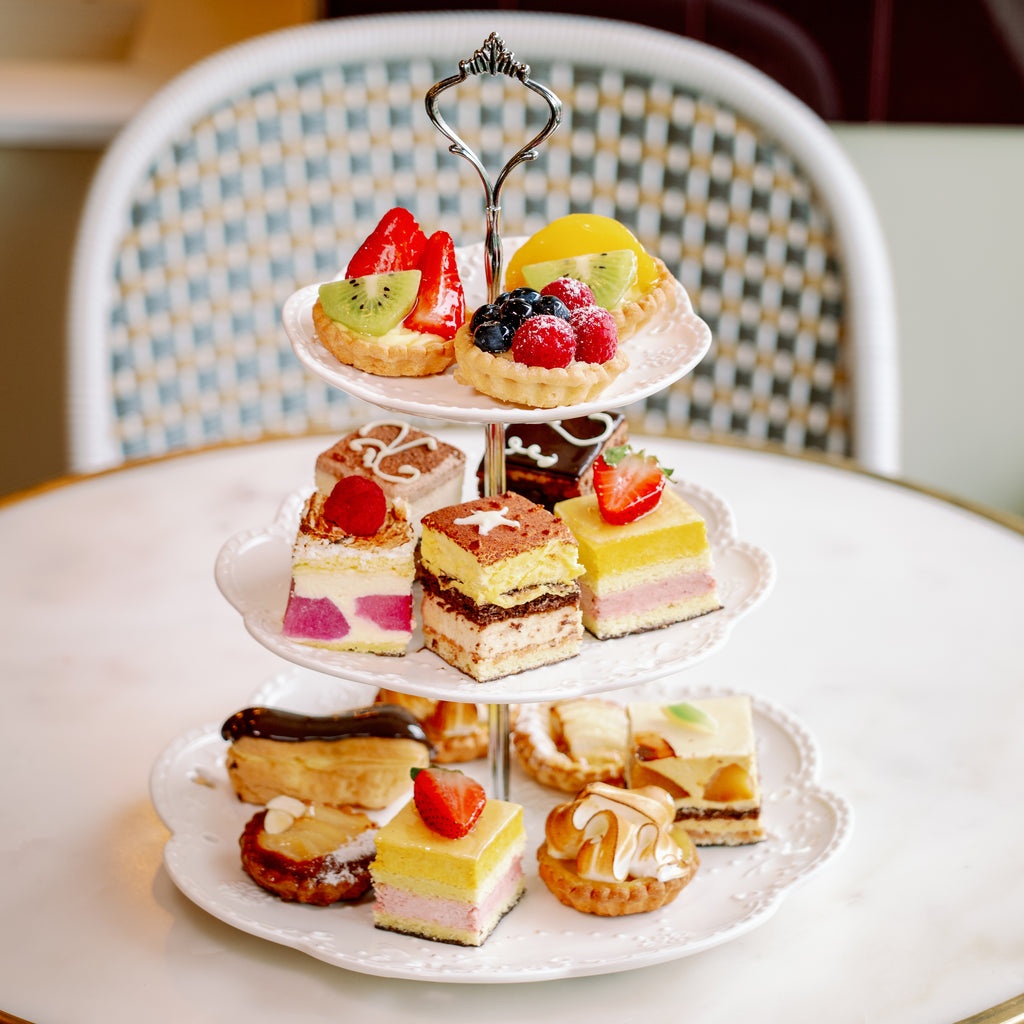This indoor close-up photograph captures a three-tiered dessert carousel, meticulously arranged on a round, plain white table. The carousel, made of white porcelain and held together by a chrome stem with a metal hook on top, showcases an array of delectable treats. The bottom and largest tier brims with a diverse assortment of cakes and baked goods, including an éclair, a fruit bar, and a miniature meringue pie. Fresh strawberries adorn some pieces, adding a dash of color. The middle tier, slightly smaller, displays an assortment of small cakes, consisting of five different desserts, likely including lemon meringue pie, cheesecake, and perhaps some chocolate truffles. The smallest and top tier holds three delicate fruit tarts, featuring fresh fruit such as kiwi, strawberries, and bananas. Each dessert is crafted with exquisite detail, some topped with chocolate or fudge for added indulgence. In the blurred background, a chair with a woven checkerboard pattern in teal, gold, and white can be seen, tucked under the table, emphasizing the focus on the beautifully presented dessert tray.